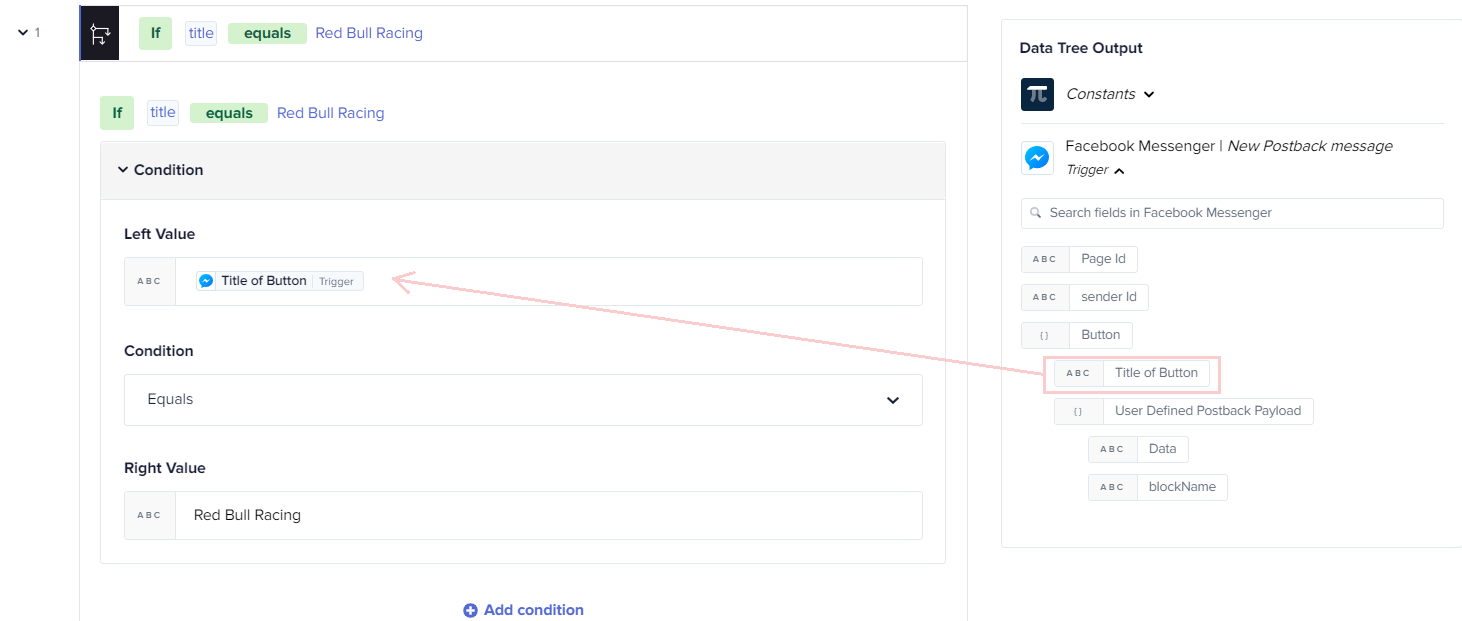The image is a detailed screenshot of an administrative panel with several conditional logic statements and highlighted UI elements. In the central portion, an "if-then" condition is displayed within a green-shaded field. The condition specifies: "If title equals 'Red Bull Racing'." Below this, a secondary conditional logic is presented with the statement: "If title equals 'Red Bull Racing', condition left value 'AMS title of button'." 

On the far right portion of the panel, there is a section outlined in a pink rectangle with a long arrow extending leftward, indicating the connection to the "left value option" under the condition. This specific element is labeled as "title of button." The condition is then defined as: "condition equals right value 'Red Bull Racing'."

Adjacent to this area, there is a data tree output displayed, characterized by a black square with rounded corners containing a pi symbol. The section is labeled "constants." Directly below this, there is a speech bubble with a blue background and a white lightning bolt icon, representing a Facebook Messenger feature. It describes the new post-back message trigger, with search fields such as "KBC page ID" and "server ID." The same section includes a reference to a "button."

Further below, while some text remains unreadable, the bottom-most part of the panel reveals a blue text with a plus sign, inviting the user to "add condition."

This screenshot appears to illustrate the setup of complex conditional logic within an administrative interface, highlighting specific configurations and UI elements pertinent to Red Bull Racing's title-related conditions.